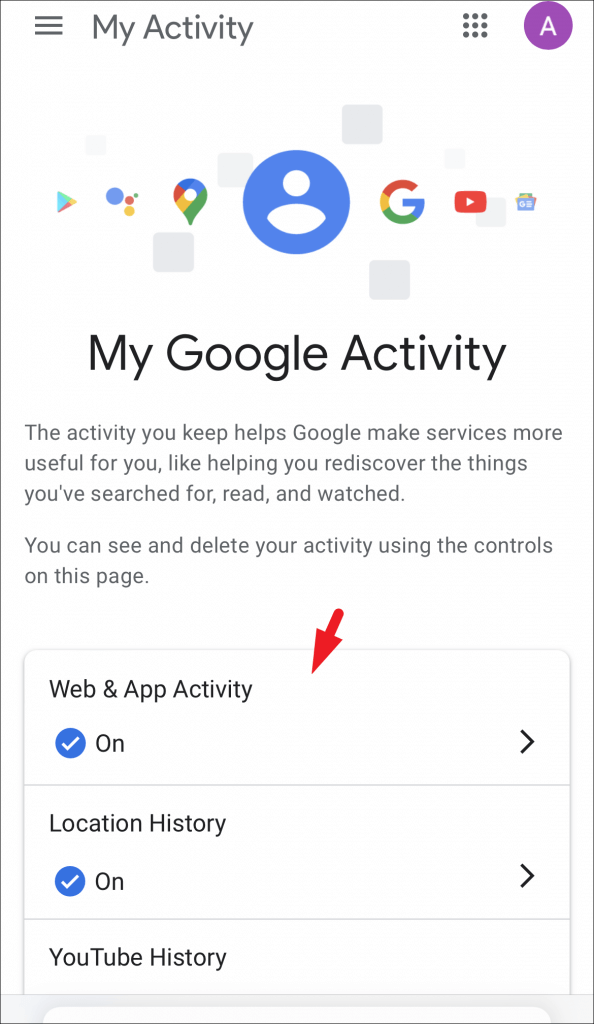A screenshot of a smartphone displaying the Google 'My Activity' web page. At the top left corner, a hamburger menu icon is visible, followed by the 'My Activity' title. Adjacent to it is a grid of nine dots, alongside a square icon, and a purple circle encasing the letter 'A'. Beneath this, a series of gray icons represent various Google services: Google Play, Maps, Google Search, YouTube, and Calendar. 

Central to the screenshot is a placeholder for the user's profile picture, under which 'My Google Activity' is reiterated. Below this, a text block explains, "The activity you keep helps Google make services more useful for you, like helping you rediscover the things you've searched for, read, and watched. You can see and delete your activity using the controls on this page."

A red arrow directs attention to three highlighted sections:
1. 'Web & App Activity' - indicated as active with a checkmark and a right-facing arrow.
2. 'Location History' - also marked as active with a right-facing arrow.
3. 'YouTube History' - partially visible, leaving it unclear if it is active or has an arrow.

The comprehensive layout provides a clear and structured view of the user’s activity settings on Google's platforms.